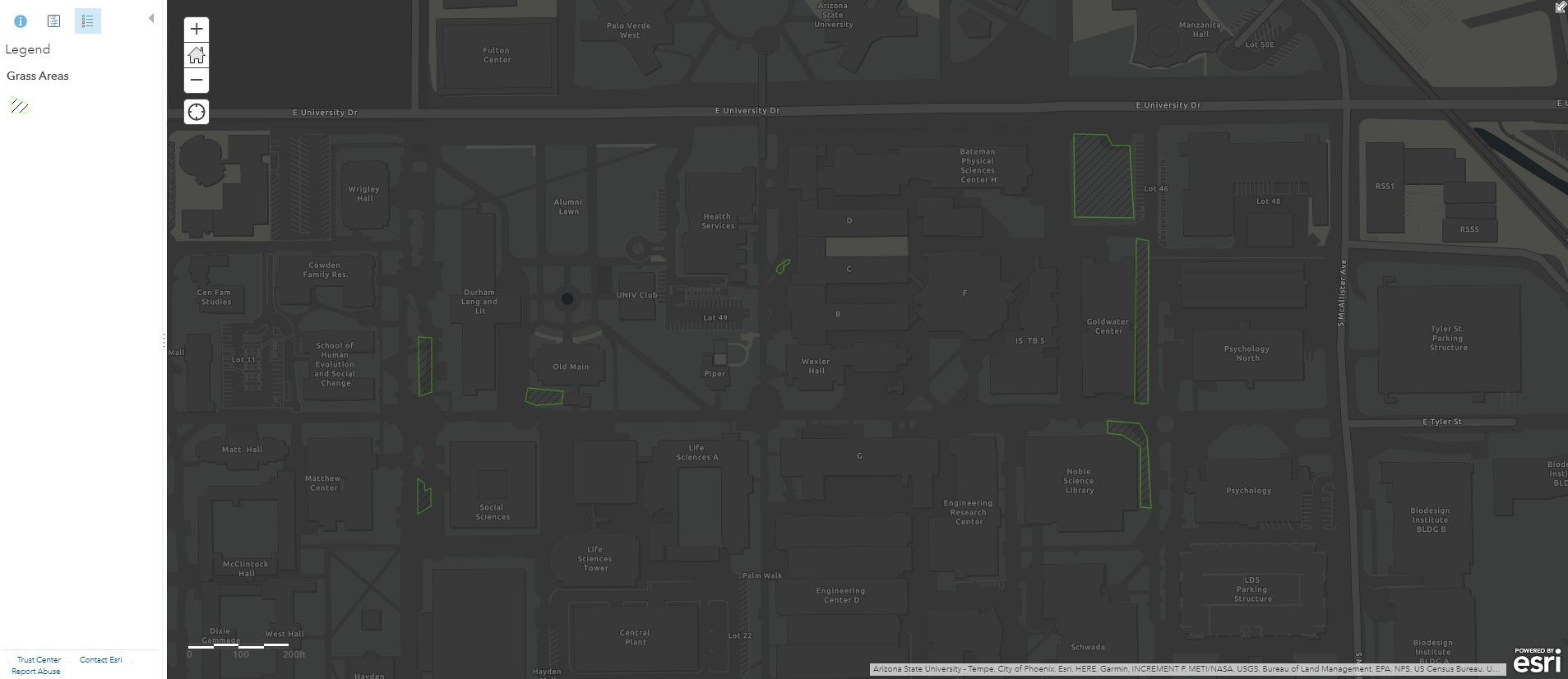The image depicts an aerial view map of an urban area, potentially a campus or a section of a town, spanning approximately eight square blocks. The map is dark with predominant hues of dark green and light green, accented by small yellow outlines. In the lower corner, the letters 'ESRI' identify the map's creator. The depiction features several large buildings interspersed with open spaces, likely parking lots. Streets crisscross the view, organizing the layout. While there are textual labels indicating the names of buildings and streets, they are too small to be legible from the current perspective. The overall impression of the map is similar to what one sees on a Google map, providing a detailed, bird's-eye layout of the area.